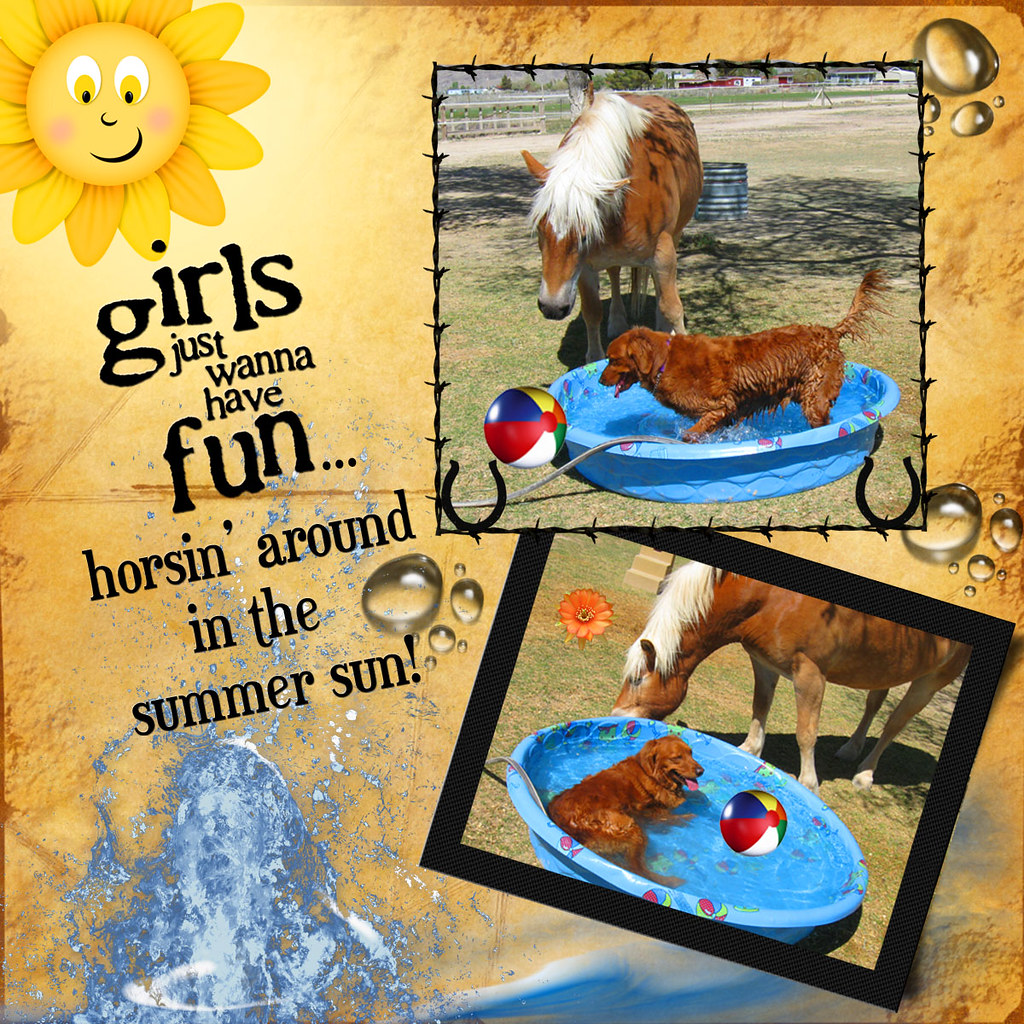The image features a creatively designed brown background reminiscent of an old map, adorned with thematic embellishments. On the upper left, a cheerful, cartoonish yellow sun with a face beams down, accompanied by the playful black text, "Girls just want to have fun horsing around in the summer sun." Below this, a splash of crystal blue water emerges from the lower left, contributing to a summery ambiance. 

On the right side of the image, there are two smaller pictures prominently displayed. The top picture captures a reddish-brown dog inside a blue kiddie pool while a brown horse with a white mane stands beside it, watching curiously. The dog's tongue is playfully out, seemingly enjoying the cool water. In the bottom picture, the same horse continues to keep company with the dog, who is now lying down in the pool. Scattered around are realistic-looking water droplets and additional summer-themed elements like a photoshopped beach ball and orange flowers, adding to the lively scene. The entire composition suggests a lighthearted, fun-filled day in the sun.